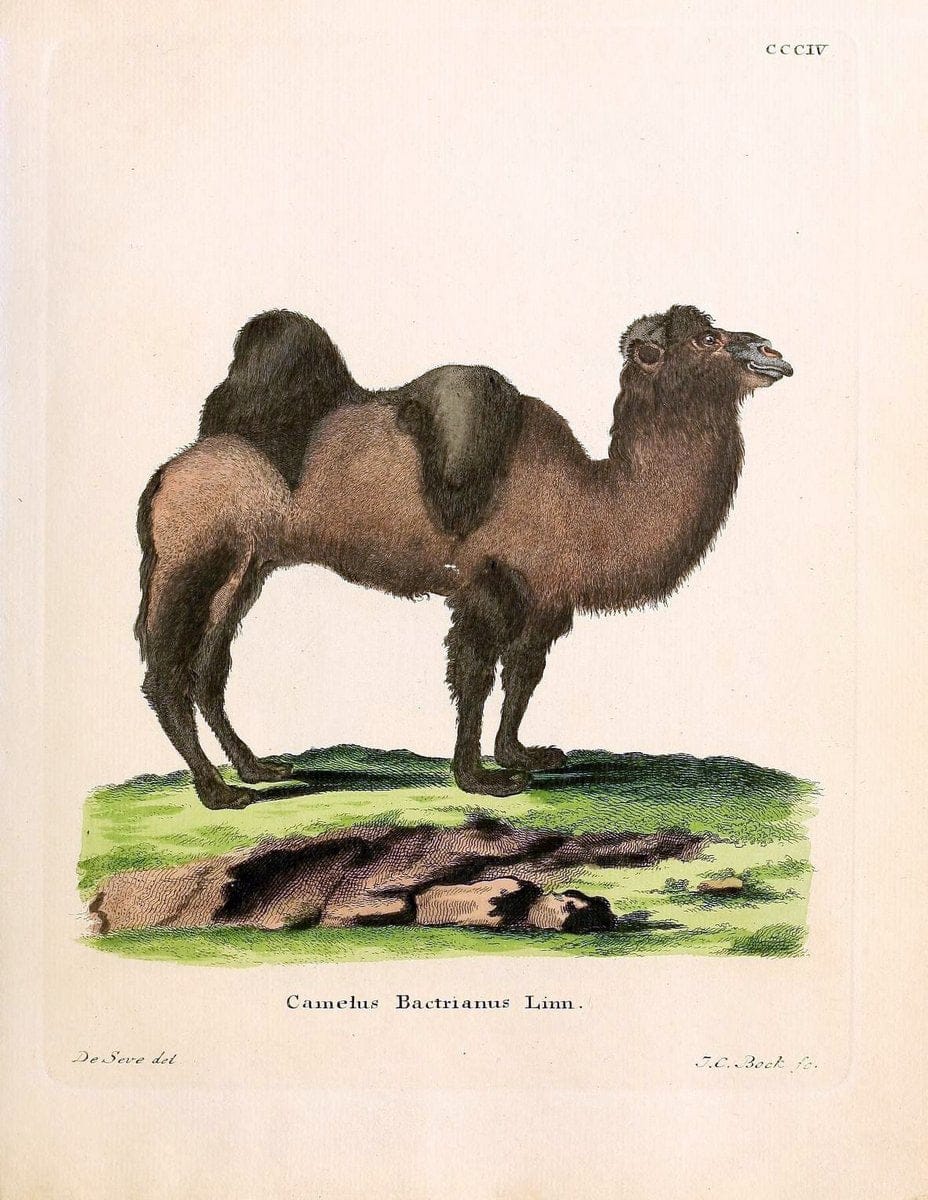This is a detailed hand-drawn illustration of a camel, facing towards the right. The camel, characterized by a long neck and somewhat peculiar features, exhibits a large, dark brown hump situated at its rear, resembling a seat in its position. The body and legs of the camel are a combination of light and dark brown, with the legs being predominantly darker. The face, slightly unconventional, has big brown eyes. The creature stands on a patch of light and dark green grass intermixed with medium brown rocks. The image is set against an ivory or beige background. Below the drawing, text reads "Camelus Bactrianus Lin."